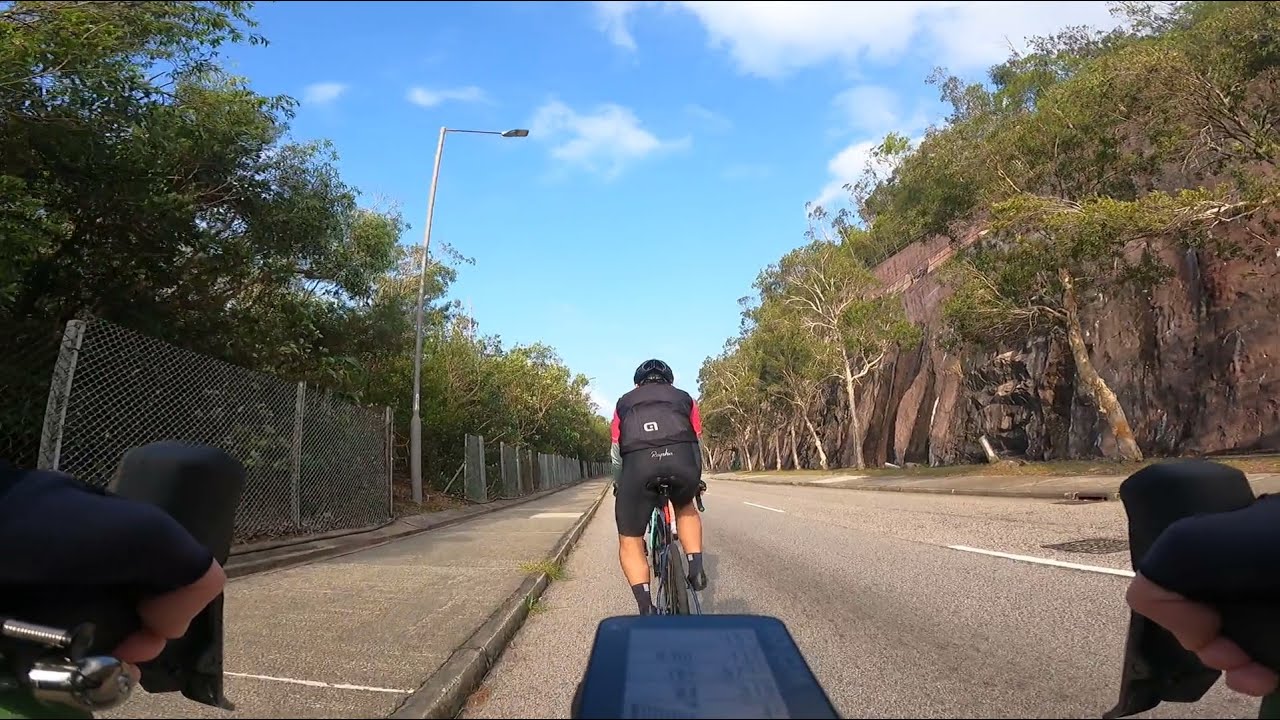From the perspective of a cyclist in a bike race, the image captures hands gripping the handlebars, adorned with fingerless black gloves, at the bottom corners of the frame. The road, a two-lane street with sidewalks on both sides, lies ahead. A black-helmeted cyclist, wearing a black backpack and black shorts, along with a red and blue striped shirt, rides directly in front, seemingly having just appeared in the scene. Their bicycle features a slight red detail beneath the seat. The left side of the road is lined with a broken metal fence interspersed with light poles, beyond which stand a few trees. On the right, a dramatic cliff adorned with sporadic trees rises through a rocky, green terrain. Above, the sky stretches out, blue and dotted with clouds, framing the outdoor setting of this intense bike race.